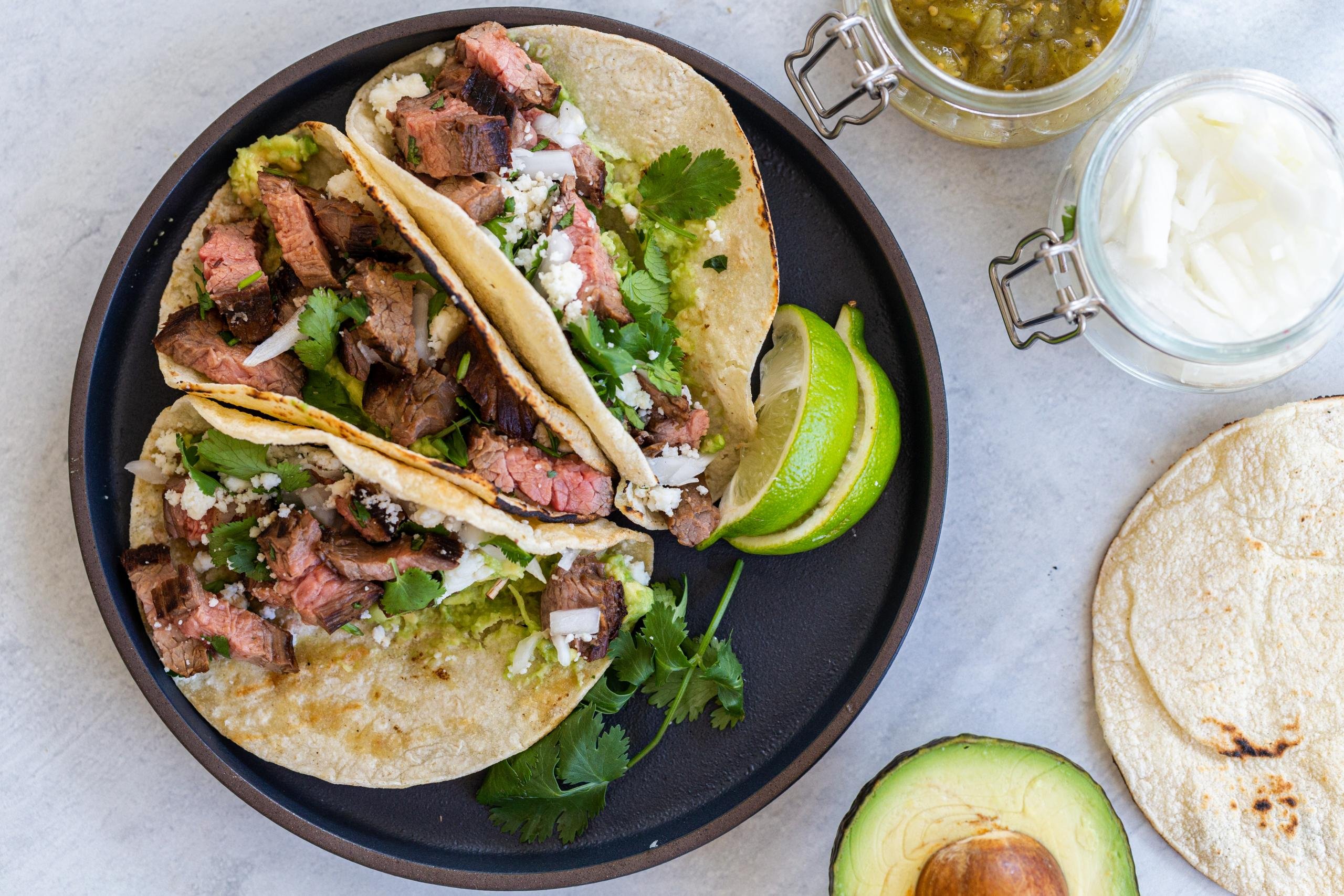This professional, overhead shot of a black plate showcases three authentic Mexican-style tacos filled with carne asada, garnished with crumbly cheese, fresh cilantro, diced onions, and an avocado mixture. The tacos are wrapped in soft flour tortillas and accompanied by lime wedges. Surrounding the plate, on a white table, are two containers—one with a greenish spicy salsa and another with sour cream. Nearby, there's a single plain tortilla and half of an avocado with the pit still intact. The setup, complete with its meticulous arrangement, looks like it belongs on the cover of a food magazine, exemplifying the essence of Mexican cuisine.